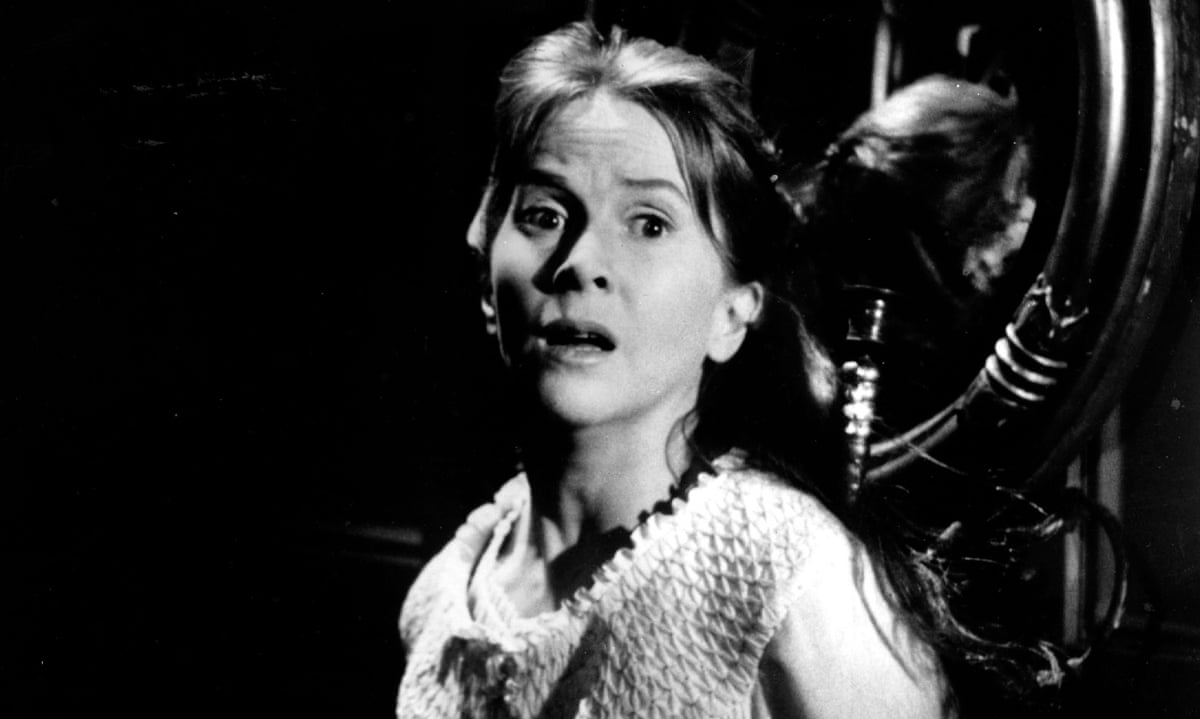The image is a black-and-white still that appears to be from a movie or theatrical play, capturing a fair-skinned Caucasian woman in a startled or fearful state. Her expressive facial features include wide, raised eyebrows and an open mouth, with pronounced creases on her forehead. She is facing the viewer directly, with her hair tied up, and there's a shadow cast on one side of her face, enhancing the dramatic effect. She wears a textured white shirt adorned with triangular patterns across the front. The background is predominantly black, making the woman's alarmed expression the focal point of the image. Behind her are three metallic rings, two of which are large and positioned near her head, with a smaller one closer to her shoulder, all appearing somewhat abstract against the dark backdrop.